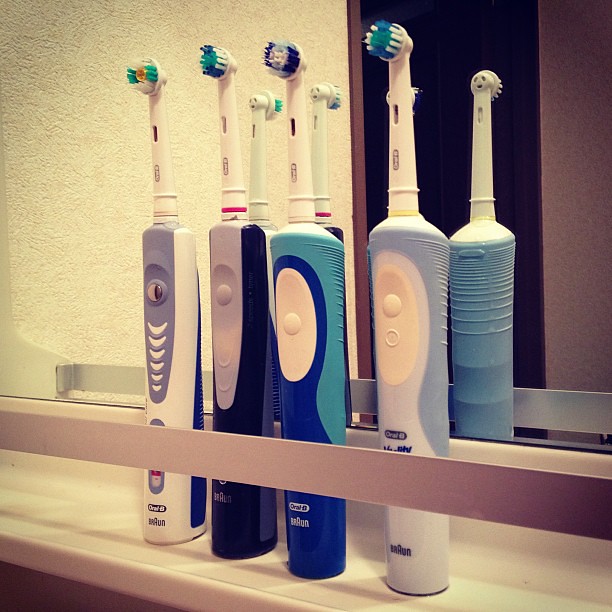This detailed image captures a collection of four electronic toothbrushes, all with circular brush heads, mounted on a sleek white platform equipped with a silver bar for secure placement. They are positioned in front of a large bathroom mirror, reflecting a white stucco side wall. Each toothbrush is distinctly colored and bears the Oral-B Braun label. Starting from the left, the first toothbrush is purple and white, featuring teal, orange, and white bristles. The second is a combination of black and light pink, adorned with white, teal, and blue bristles. The third toothbrush is dark blue with a teal blue accent and has bristles in shades of white, teal, and blue. The final toothbrush on the right is light blue and white, equipped with similar-colored bristles. The bathroom's background details include a stucco wall and possibly a marble-like counter that provides a polished and structured ambiance to the scene.